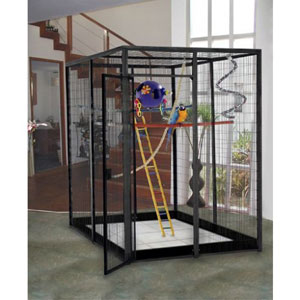The image features a large black metal birdcage, resembling an aviary, with a white floor and positioned on a gray concrete floor. The door to the birdcage is open. Inside the cage, there's a yellow ladder and a purple object situated in the middle. Perched on a red peg is a relatively large bird with blue and yellow plumage. The backdrop of the scene includes a spacious room with a tall window trimmed in white, letting in natural light, and a spiral staircase leading to an upper level. The birdcage is set against this window, and nearby, there seems to be additional greenery enhancing the indoor environment.